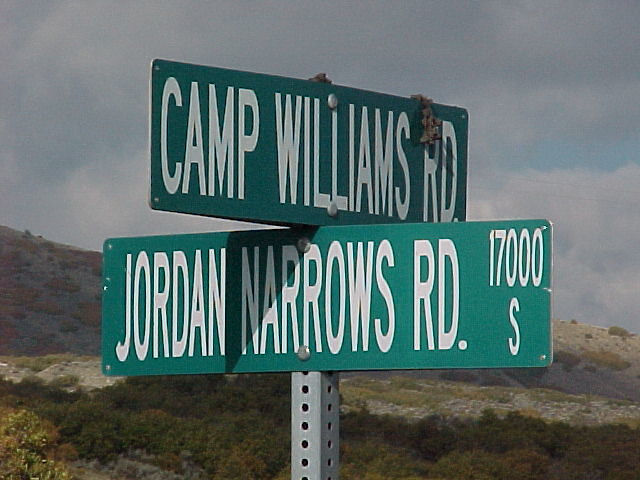The image captures a detailed view of a road intersection sign set against an overcast sky, with patches of blue breaking through the gray. In the background, rolling hills dotted with shrubs and lots of exposed dirt suggest a dry, arid climate. The intersection sign comprises two green panels on a silver post. The top panel, partially obscured by brown vegetation, reads "Camp Williams Road" in white letters and is oriented away from us. The bottom panel, facing us directly, reads "Jordan Narrows Road, 1700 South." The shadow of the top sign overlaps the "N" and "A" in "Narrows," adding depth to the image. Additional vegetation is visible below the signs, blending with the rugged, dry landscape.